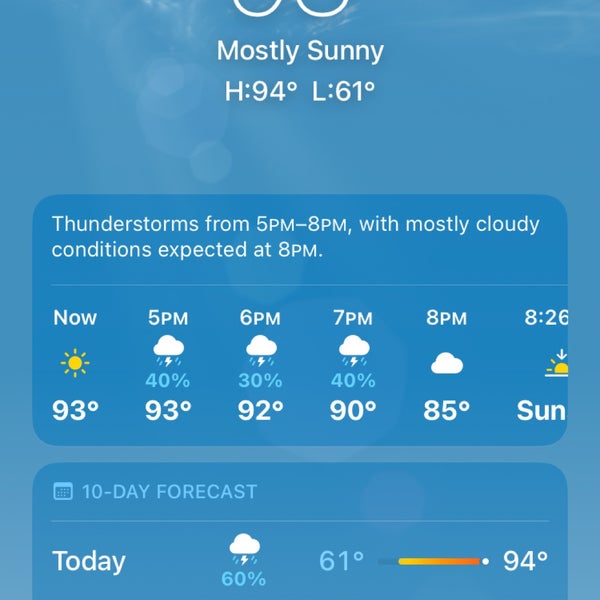This image appears to be a screenshot of a weather application or widget. The background is a soothing light blue, resembling the color of the sky. The top portion of the image is slightly cut off, but you can still see some white semicircles in the middle, giving the impression of a weather icon. Below these semicircles, the text "Mostly Sunny" is displayed in white font.

Underneath this, the temperature highs and lows are listed: "H: 94°F, L: 61°F." Further down, a prominent horizontal box in a darker shade of blue provides additional weather details: "Thunderstorms from 5 p.m. to 8 p.m. with mostly cloudy conditions expected at 8 p.m." 

Below this, hourly updates from "Now" to "8 p.m." are listed. These updates include temperatures and weather conditions:
- 5 p.m.: Cloud icon, 93°F, 40% chance of rain.
- 6 p.m.: Cloud icon, 93°F, 30% chance of rain.
- 7 p.m.: Cloud icon, 92°F, 40% chance of rain.
- 8 p.m.: Cloud icon, 90°F, 0% chance of rain.
  
The progression of temperatures continues with the last entry at "8:26 p.m.," displaying 85°F and a sun icon next to it.

Towards the bottom, there’s another box with a "10-day forecast" labeled in light blue. Directly under this, in white text, it says "Today" with a white cloud icon and "60%" next to it, indicating precipitation probability. Adjacent to this, the temperatures are listed again: "L: 61°F" and "H: 94°F." An orange to dark orange gradient bar represents the temperature range for the day.

This detailed weather app screenshot offers a thorough and visually organized overview of the current and upcoming weather conditions.